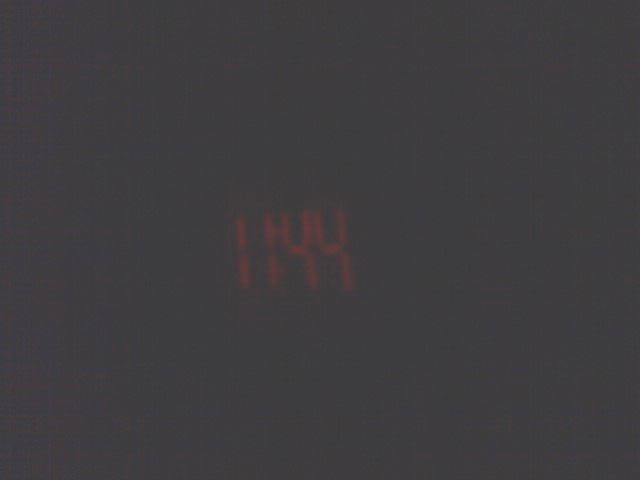In this image, the scene is predominantly composed of dark gray tones, reminiscent of a photo taken in a nearly pitch-black room. Dominating the center of the frame are the faintly glowing red digital numbers "1144," which appear to be from an alarm clock or similar device. The numerals are constructed from segments, typical of digital displays, and seem to be viewed from a slight angle, as the numbers appear slightly smaller on one side. The background is a dark charcoal gray, and there are no other discernible objects or features in the frame. The display itself is not very clear; both the numbers and the surrounding area have a blurred, somewhat indistinct quality, making the digits blend slightly into the murky backdrop.